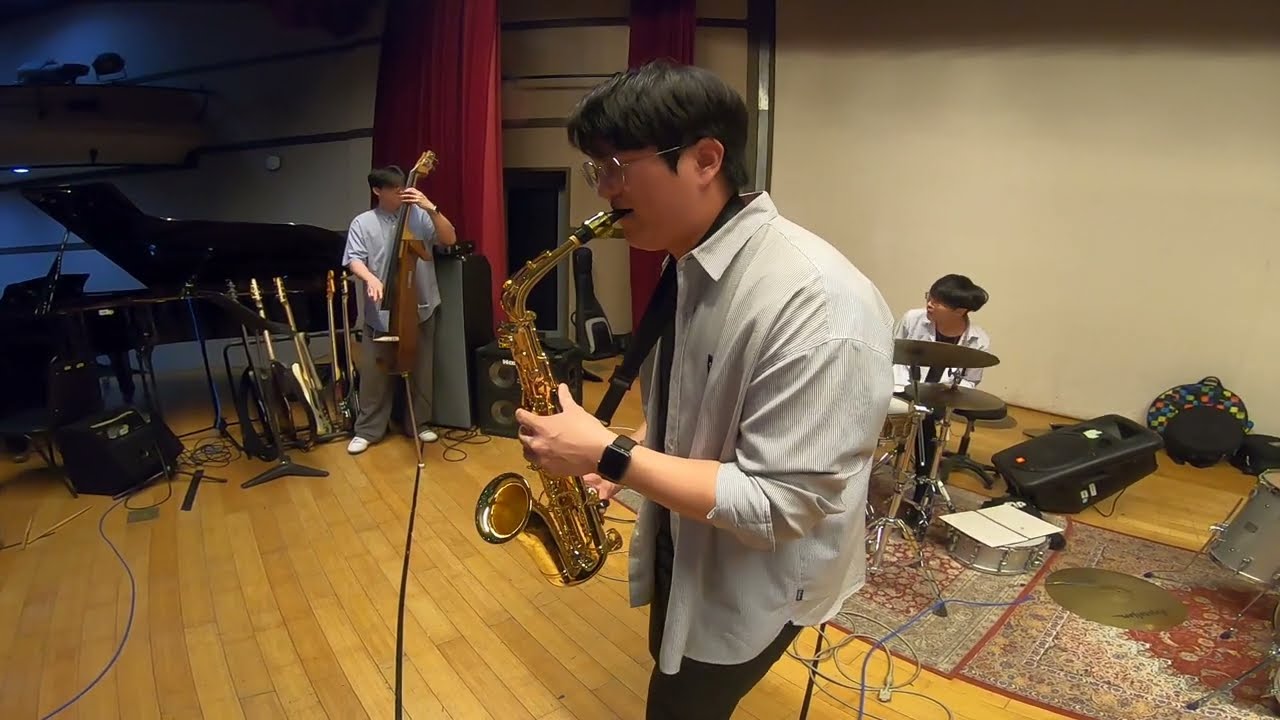The detailed description of the image brings together the shared details from the different captions:

The image depicts a band practicing indoors on a stage, likely within a gymnasium or auditorium. The band consists of three Asian individuals with short black hair, each playing an instrument. In the front and center is a man wearing glasses and a gray shirt, playing a saxophone. He sports a black smartwatch on his left arm. Behind him on the left is another man standing with a guitar held vertically; several other guitars and an amplifier are visible next to him. Situated further back and to the right is a female with her hair in a bun, wearing glasses and a white shirt, playing a drum set. The drum set is placed on top of light and dark red Persian rugs. The floor is light hardwood, and the backdrop includes large red curtains, adding to the impression of an indoor stage setup.